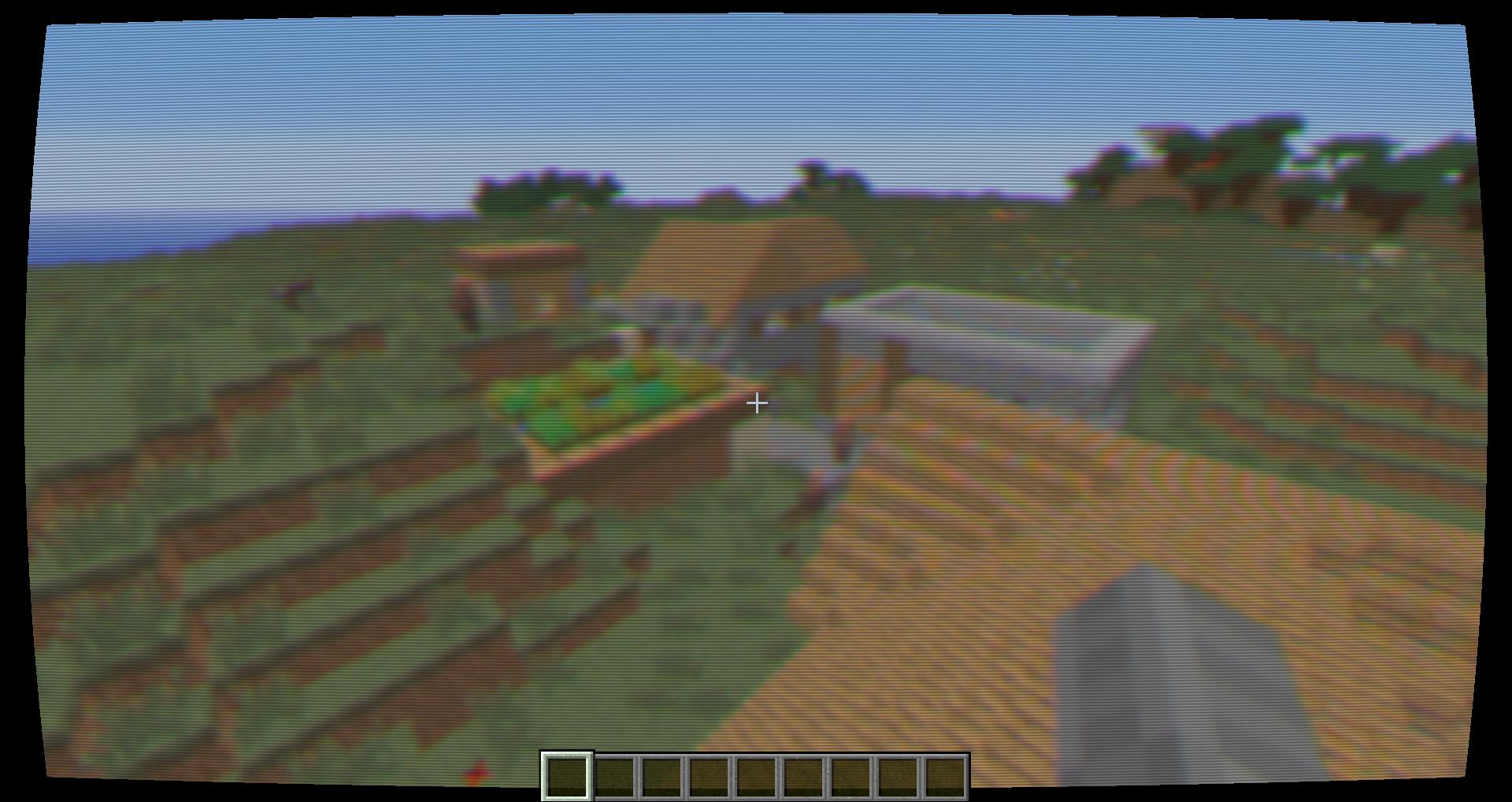This image is a screenshot from a computer game, likely Minecraft, characterized by its distinct pixelated graphics. The scene is framed by a slightly rounded, black border reminiscent of an old television screen. The pixelated graphics depict a serene landscape of grassy terrain interspersed with small, jagged hills. Several houses, constructed from grey blocks with brown roofs, dot the landscape. In the distance, a clear blue sky meets the sea, adding depth to the scene. Along the bottom of the image, black squares serve as in-game infographics, providing essential game information to the player.